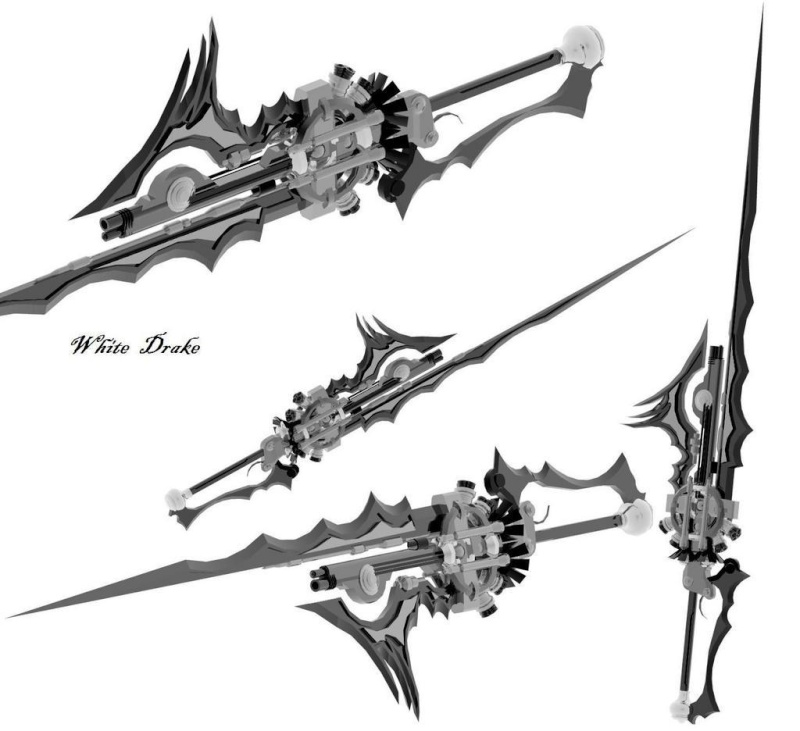The image features four silver and gray objects with sharp blades, displayed against a white background. The only text visible in the image reads "White Drake." The objects are long, slender, and feature complex designs, possibly incorporating gears and moving parts. While they resemble weapons or tools, their exact purpose is unclear. Three of the objects are positioned horizontally in the middle of the image, while the fourth is oriented vertically on the right side. The bottom item appears darker gray compared to the others. The overall aesthetic suggests it could be a product image, potentially from a website, showcasing these intricately designed items.